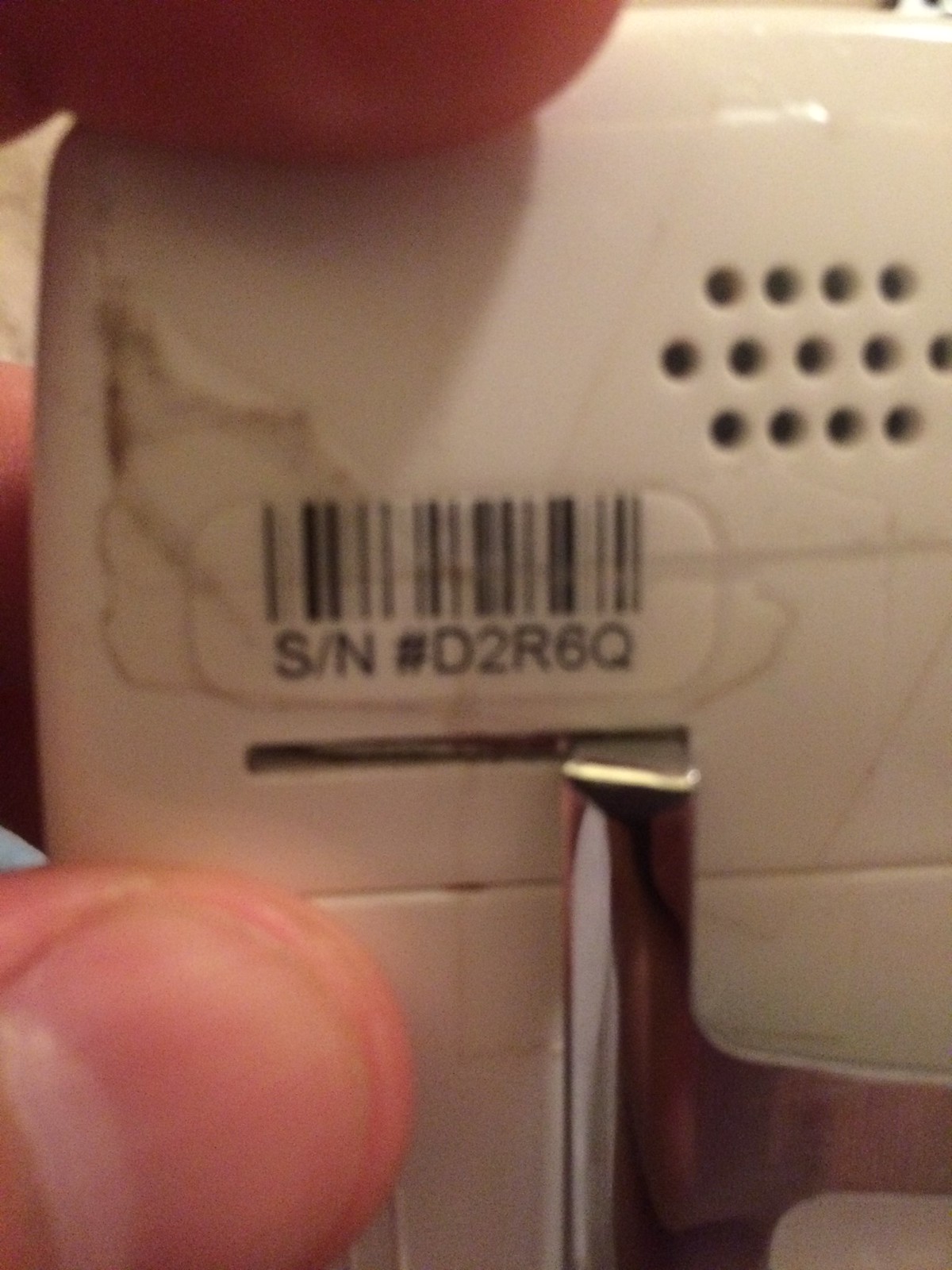The image features a white device that appears to be part of a retail or inventory system. At the center of the device, there is a rectangular label with a barcode designed to be scanned at a store. Underneath the barcode, there is a text S/N: D2R6Q written in black ink. The label is affixed to the surface of the device, which seems to be made of white plastic.

In the upper right corner of the device, there are several small black holes that resemble a speaker or ventilation grid. Above this area, two fingers are visible: the index finger positioned at the top left and the thumb positioned at the bottom right, possibly indicating someone holding or interacting with the device. Below the label, there is a small horizontal slit with a metallic component protruding slightly from it.